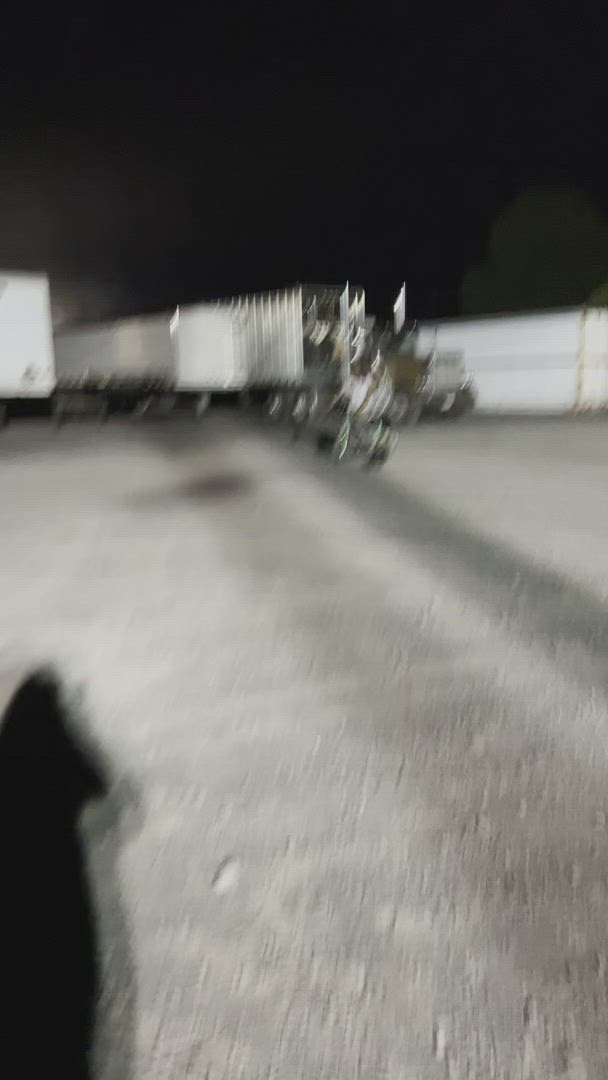In this nocturnal, portrait-oriented photograph, a sense of mystery and motion pervades the scene. The image suffers from significant blurriness and lack of focus, adding an element of intrigue. Dominating the frame's top third is an expanse of deep black, indicating the time of night. The bottom two-thirds reveals a white cement surface, likely a parking lot. Lending a human touch to the composition is the shadow of an individual, presumably the photographer, situated in the bottom left-hand corner. 

In the hazy background, a series of indistinct, white, and chrome-colored shapes vaguely suggest the presence of trucks. Some of these shapes feature a mix of horizontal and vertical white lines, enhancing the image's sense of dynamic motion. Despite the extreme blurriness, the photograph manages to evoke an atmosphere of an active, albeit enigmatic, nighttime environment.